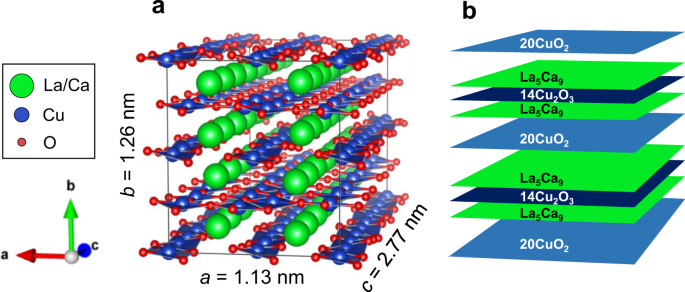The image is a detailed scientific chart divided into four sections. On the far left, a legend is displayed inside a white box with a black outline. It contains three colored dots: a large green dot labeled "La/Ca," a medium blue dot labeled "Cu," and a small red dot labeled "O." Below this, three arrows—red, green, and blue—are connected, each pointing in different directions (left, up, and right, respectively) to illustrate 3D spatial axes.

Adjacent to the legend on the right, Section A depicts a cluster of green, blue, and red balls representing a chemical structure. The green balls (La/Ca) are mostly isolated, while the blue (Cu) and red (O) balls are interconnected. This section includes diameter measurements of the clusters, specifying the dimensions as 1.13 nm by 1.26 nm by 2.77 nm.

To the right of Section A, Section B features a series of flat, paper-like layers colored in shades of blue and green. Each layer is inscribed with chemical formulas, such as "20CuO2," indicating different compositions.

Overall, the chart visually represents chemical configurations and spatial dimensions, highlighting intricate details across its sections.